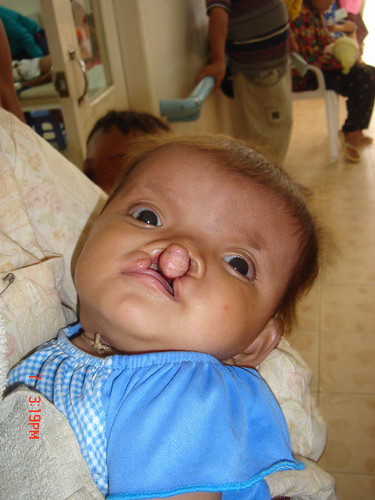The photograph captures a baby with a cleft lip, lying in the arms of a woman who is wearing a light, flowery button-down shirt. The baby, with light brown skin and hair, is dressed in a blue outfit featuring a light blue checkered pattern on the front. The cleft lip and the associated facial deformities, including a gap between the nose and mouth and widened eyes, are prominently visible. The background setting appears to be a hospital, indicated by the presence of multiple people, some with injuries. Flooring is a yellowish square tiling, and the wall towards the center-top is painted white with a long, blue painted metal railing. In the top left corner of the image, a double door with glass panels is partially open. The photograph also includes an orange timestamp reading "1:19 PM" superimposed on the right side.